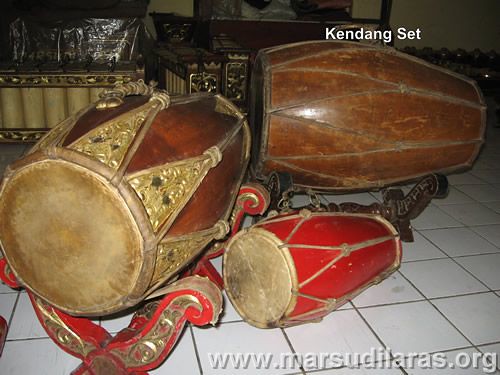The image features a set of three traditional drums, likely of African origin, placed on a white tiled floor. The drums are laid on their sides, with the background showcasing some wooden furniture. Each drum is detailed and intricately designed. The two larger drums have deep brown wooden barrels, aged with a rich patina, and their drumheads are crafted from dark, worn leather. They feature metallic triangular highlights on the sides extending from the drumhead to the barrel. The smaller drum stands out with its vibrant red barrel, brown top, and tan strings securing the drumhead in place. This drum, like the others, exhibits a special design with strings that contribute to its structure. Additionally, the top of the rightmost drum bears the white inscription "Ken Duncan set." At the bottom of the image, there is a website link in white or light grey text that reads "www.masutilaras.org," adding a modern element to the traditional aesthetic of the scene.